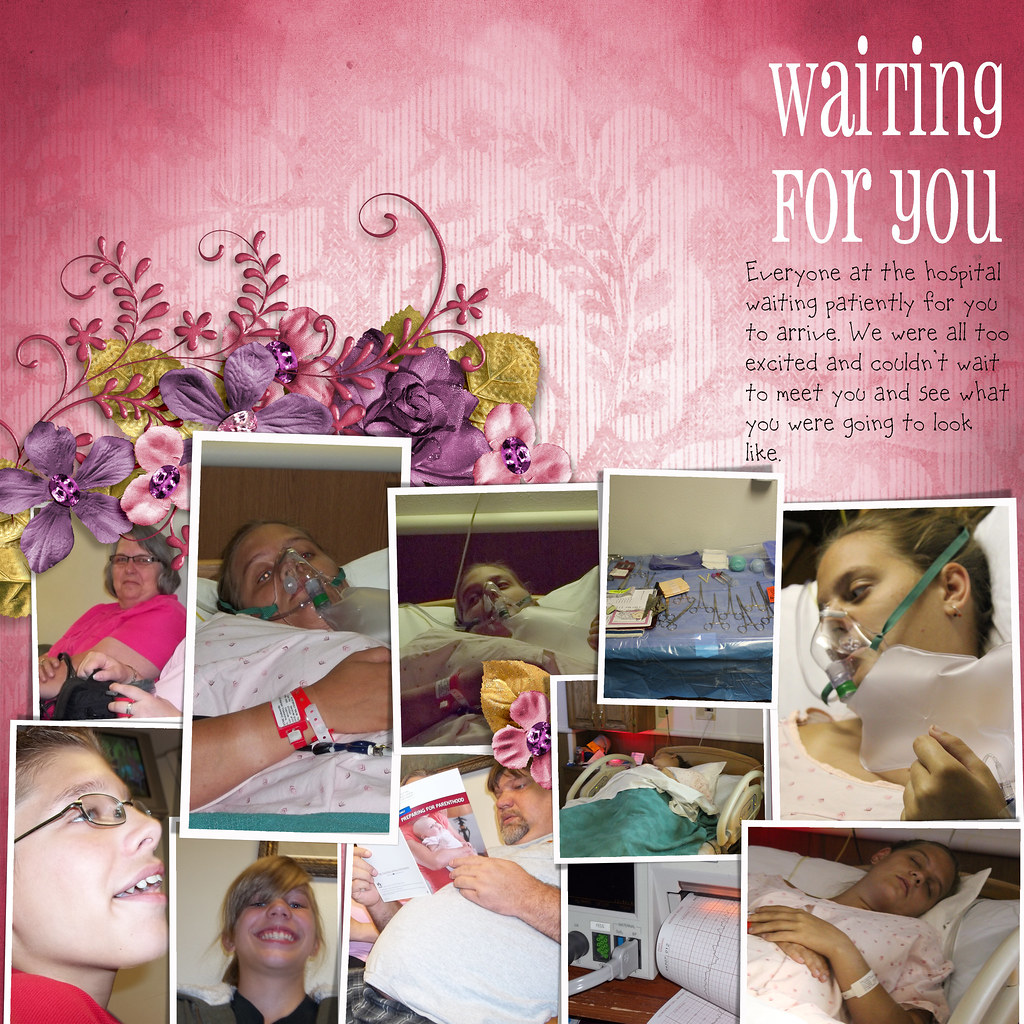This digital image features a pink background adorned with flower patterns. On the top right, the text "waiting for you" appears in white lowercase letters. Beneath this heading, in black font, it reads: "everyone at the hospital waiting patiently for you to arrive, we were all too excited and couldn't wait to meet you and see what you were going to look like." The lower half of the image showcases a collage of several pictures, including Polaroids. These images depict a variety of scenes: a person lying on a hospital bed with an oxygen mask, a man sitting in a chair reading a book about a child, a grandmother with gray hair, and several selfies of people in both hospital and normal settings. This evocative collage appears to capture moments of anticipation and emotion among family and friends at the hospital.